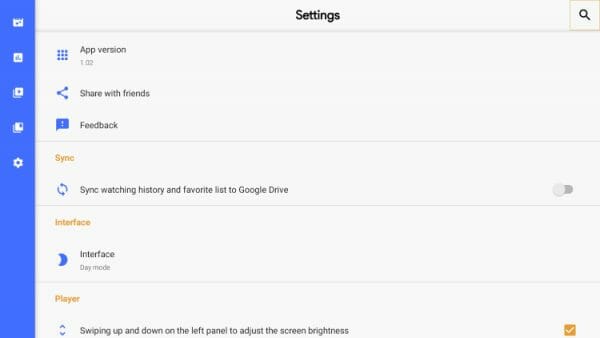The image depicts a detailed settings screen. At the top, there's a light grey panel with the word "Settings" prominently displayed in bold in the center. On the right side of this top panel, there's a magnifying glass icon meant for search functionality.

Running vertically along the left side is a blue banner featuring various icons that represent different settings categories. Adjacent to this banner, on the right side, are additional icons and categories available for selection.

The first panel includes options such as "App Version," "Share with Friends," and "Feedback," each accompanied by its respective icon. For instance, the icon for "App Version" resembles a grid of squares, while "Feedback" features a speech bubble with a question mark inside.

The second panel highlights the "Sync" option, displayed in orange. It states, "Sync watching history and favorite list to Google Drive," with a circular refresh icon next to it. To the right of this, there is an enable/disable toggle, which is currently set to disabled.

Below that, the next highlighted panel shows "Interface" in orange. Further down is the "Player" section, also in orange, which explains that swiping up and down on the left side of the screen adjusts brightness. An orange checkbox is situated to the right of the "Player" panel, indicating that this feature is currently enabled.

This detailed visual layout allows for easy navigation and customization of the application's settings.